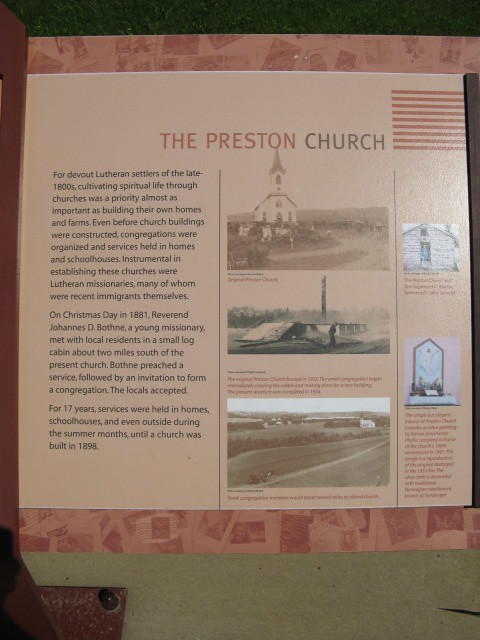The image depicts an informational sign, possibly part of a museum exhibit, detailing the history of Preston Church. The sign has a white or off-white background with pinkish borders at the top and bottom. The title, "THE PRESTON CHURCH," is prominently displayed in a red font at the top, with "CHURCH" in black, all in capital letters. Down the left side of the sign is a column of explanatory text. This text discusses the importance of spiritual life for devout Lutheran settlers in the late 1800s, noting that cultivating their faith was almost as crucial as building homes and farms. It describes how, before church buildings were erected, congregations were organized, and services were held in homes, schoolhouses, and even outdoors during the summer months. Instrumental to this spiritual cultivation were Lutheran missionaries, many of whom were recent immigrants themselves. Specifically, it mentions Reverend Johannes D. Boffner, who preached on Christmas day in 1881, leading to the formation of the congregation. For 17 years, these early services were conducted in various locations until the church was built in 1898.

The right side of the sign features three black and white photographs. The first image shows a white church with a spire; the second photo depicts a bridge over a river with a single man standing on it; and the third image captures fields and hedgerows with a white church in the top right corner. Additional smaller images of the church are positioned on the right side of the text column, though they are too small to read in detail. The entire sign appears to be attached to a wall with a newspaper-like background surface and a green banner at the bottom.